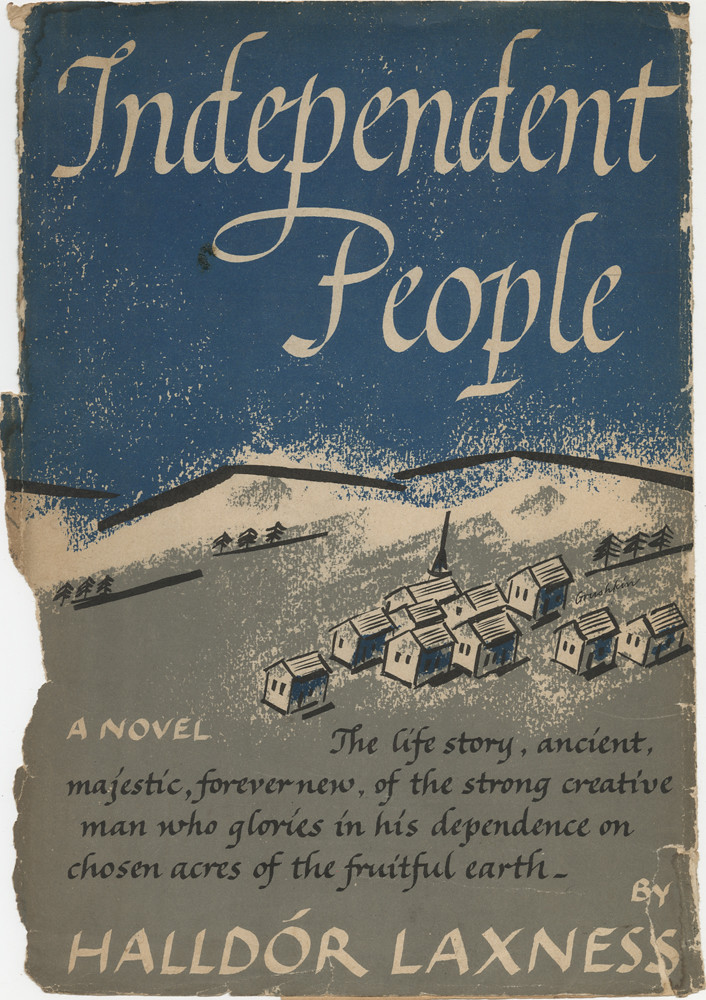This image captures the worn and tattered cover page of a novel, likely scanned or photographed. The cover features a blue night sky with white lettering at the top, reading "Independent People." Below the text, an illustration depicts a mountainous landscape adorned with trees and a small cluster of houses that resemble a quaint village. Snowcaps crown the mountain tops, and the ground is shaded in gray tones. The title of the book is complemented by a brief description in black letters, stating: "A novel, the life story, ancient, majestic, forever new, of the strong creative man who glories in his dependence on chosen acres of the fruitful earth." The author, Haldor Laxness, is credited at the bottom in white letters. The edges of the cover are jagged and ripped, indicating its weathered condition and heavy use.